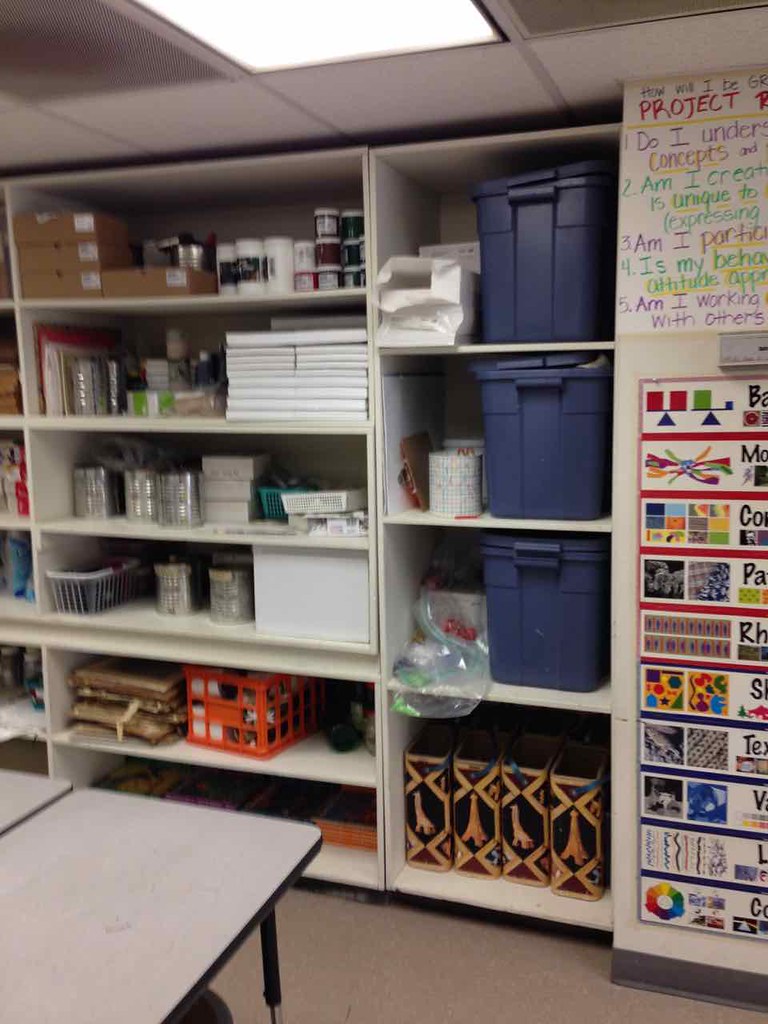The image depicts a well-organized storage room, likely used for crafts or classroom supplies, with various items meticulously arranged on white shelving units that extend from the floor to the ceiling. In the bottom left corner of the room, there are two red tables positioned side by side. The right table appears to have a store or drawer unit underneath it. On the shelves towards the right side of the image, three large blue plastic containers are prominently placed on the top three shelves. Below these containers, there are four large books, two of which feature images resembling the Eiffel Tower, and another two accompanied by tall wooden chairs. To the immediate right of these shelves, a whiteboard is mounted on the wall, displaying multicolored writing. The room is illuminated by a ceiling composed of gray panels equipped with lights. The storage shelves contain a variety of art supplies, including cans of paint, canvases, canisters filled with various colored materials, and reams of paper. The colorful decorations and posters, along with the organized storage, suggest that this room may serve as a part of a classroom or an art studio.